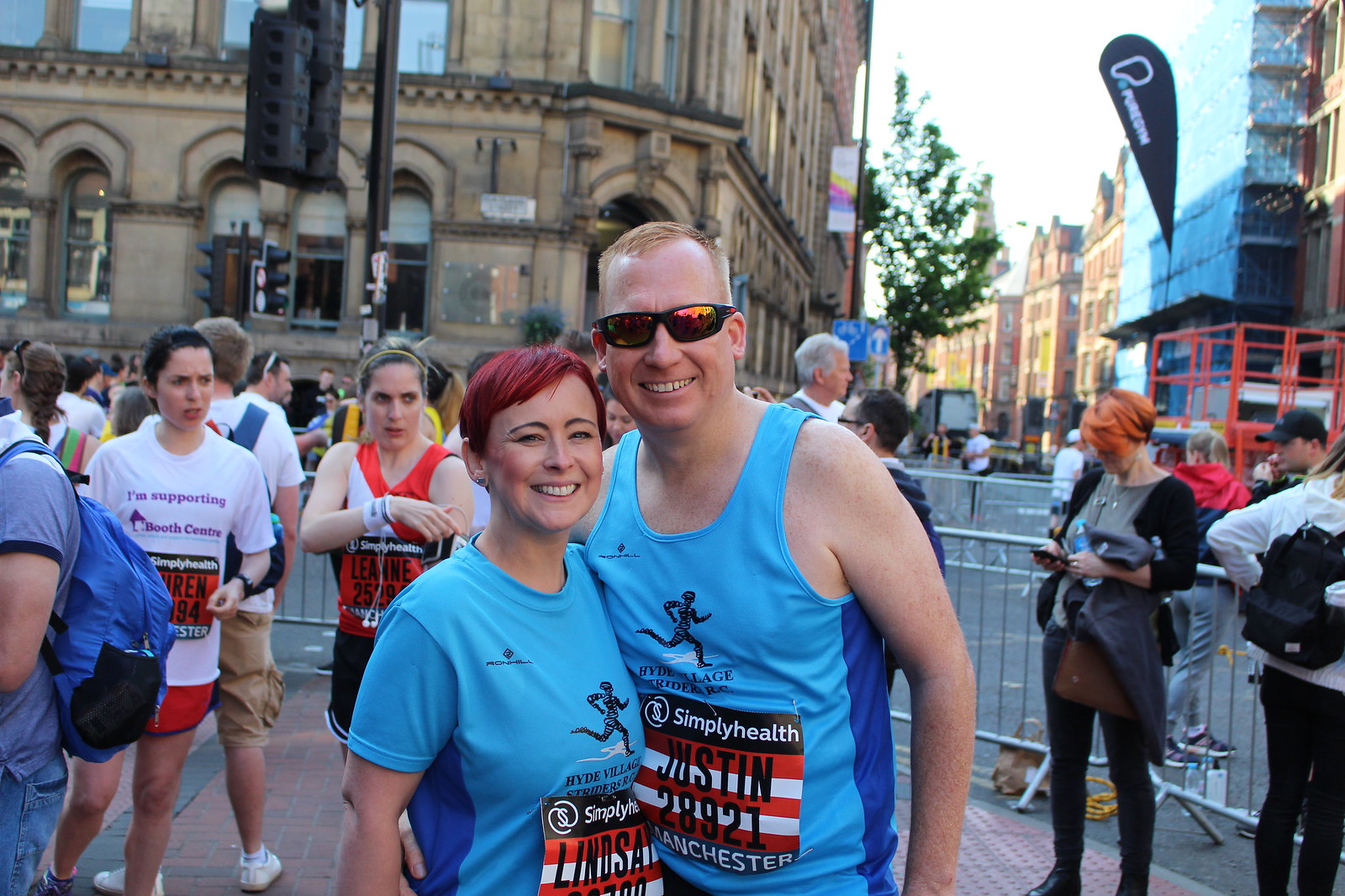In the foreground of this vibrant city street scene, a couple of marathon runners, a male and a female, stand side by side, ready to commence. The man, wearing glasses and a blue sleeveless tank top with a black runner figure, has a race bib reading "Simply Health Justin 28921." Beside him, the woman, with short red hair and a matching blue t-shirt with the same black runner figure, sports a bib reading "Lindsay," though her number is partially obscured. Behind them, a bustling crowd of fellow runners and pedestrians flanks the barricaded street, hinting at the excitement just before the race's start. The scene, dominated by a large brown stone building and a row of brick structures to the right, suggests a historical European city through which the race will traverse. Among the onlookers, a woman with orange hair dressed in all-black checks her phone, seemingly a spectator. Traffic lights mark the intersection, and a white sky stretches above, completing this detailed snapshot of an urban marathon gathering.